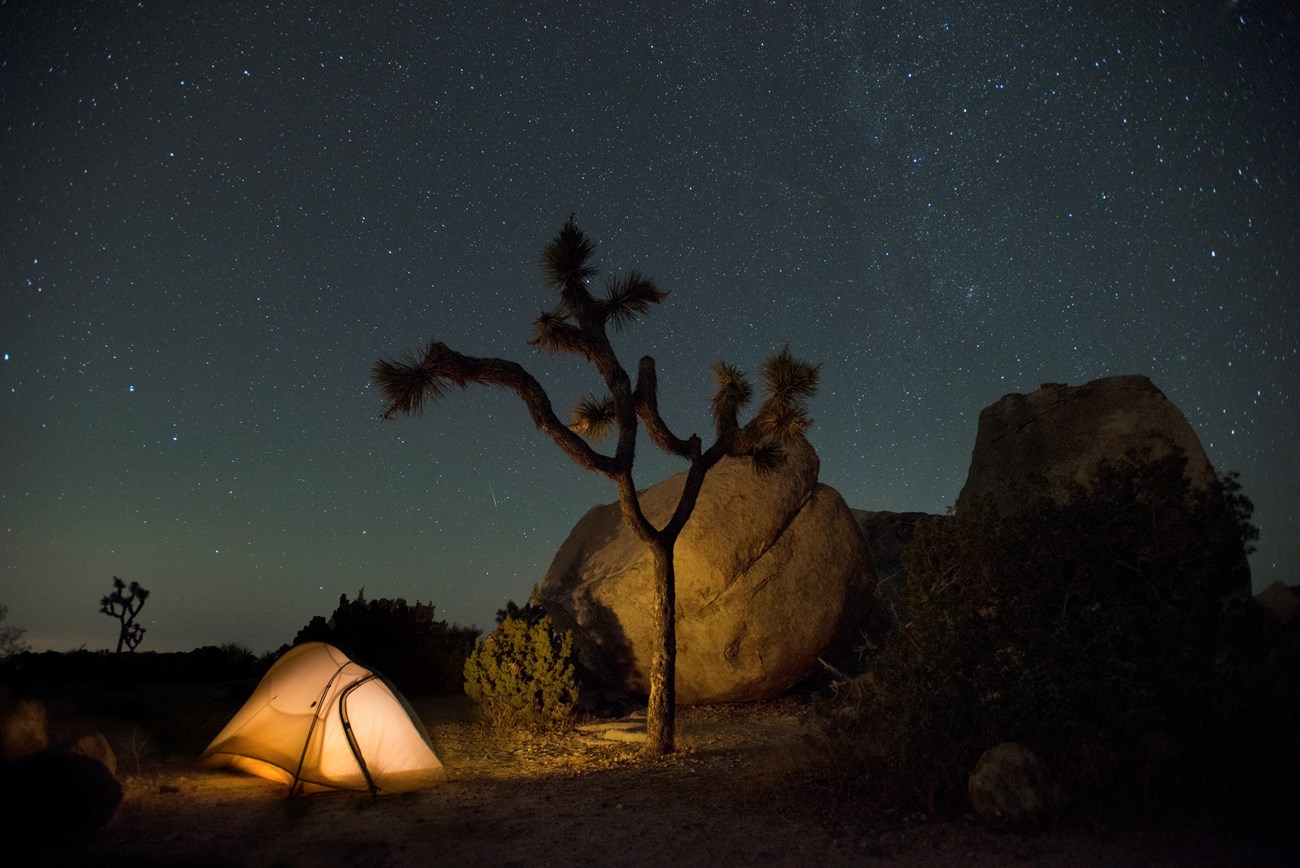A serene nighttime scene unfolds under a vast, star-speckled sky. At the center of the image stands a small tent, emanating a soft, warm glow from the light within, subtly highlighting its white fabric against the dark backdrop. The tent is pitched outdoors, nestled beside a massive boulder that dominates the foreground, its rough texture and imposing size adding a sense of rugged wilderness. Towering adjacent to the tent is a unique, leafless tree with an intricate network of branches adorned with green, prickly bush-like growth on their tips. Sparse bushes scattered around the ground complete this tranquil setting, immersing the viewer in the beauty and stillness of nature at night.